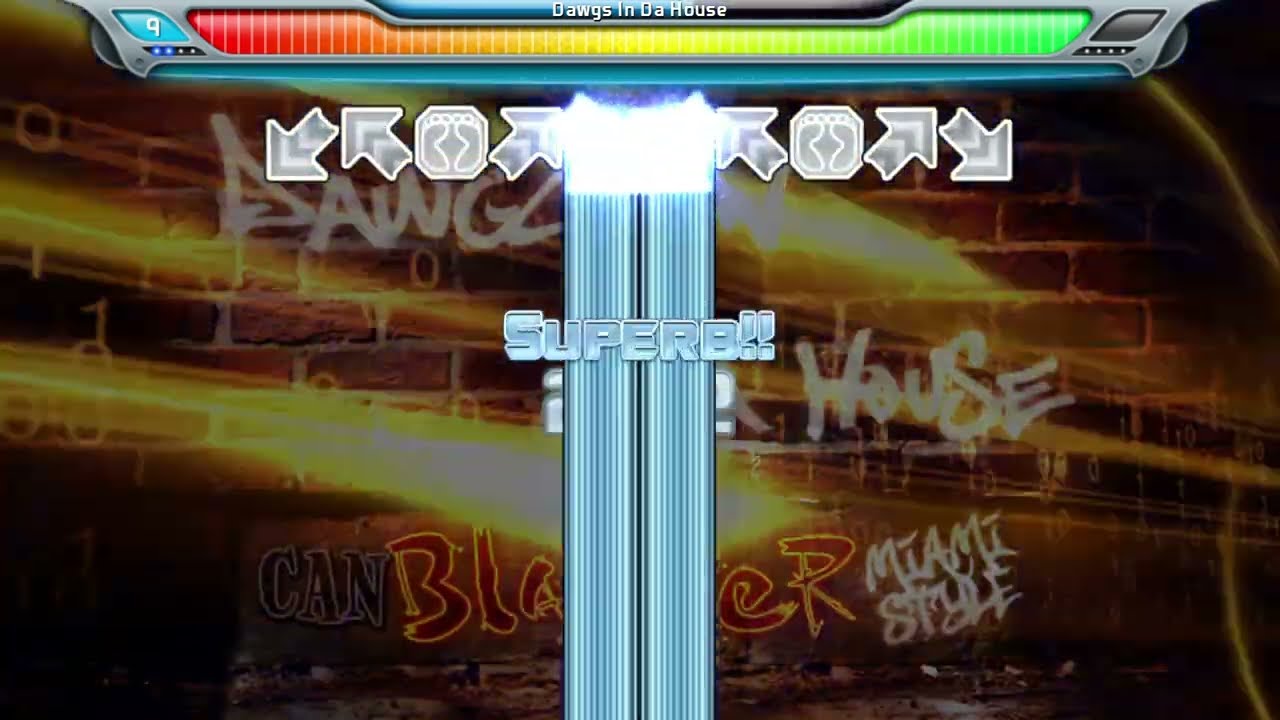This image appears to be a screen capture from a video game, possibly a rhythm or dance game similar to Guitar Hero. The background features a brown brick wall with graffiti-style writing that includes words and phrases such as "dogs," "dogs in the house," "Miami style," "can," and "blaster." At the top of the image, a control bar spans from left to right, transitioning in color from red through yellow to green, with a number 9 on the left side. Above the control bar, in white lettering, it says "Dogs in da House."

Below this, various control buttons with different directional arrows (down, down-left, up-left, up-right) and foot symbols within hexagons are displayed. These buttons are likely part of the game's interactive interface. There is also a blue column running vertically down the center of the image, with the word "Superb!!" prominently displayed in blue. The entire interface has a silver and blue design, with additional decorative elements like a silver frame around the control bar, a black strip at the top, and a blue strip at the bottom. The visual complexity and colorful elements suggest a dynamic, engaging gameplay experience.